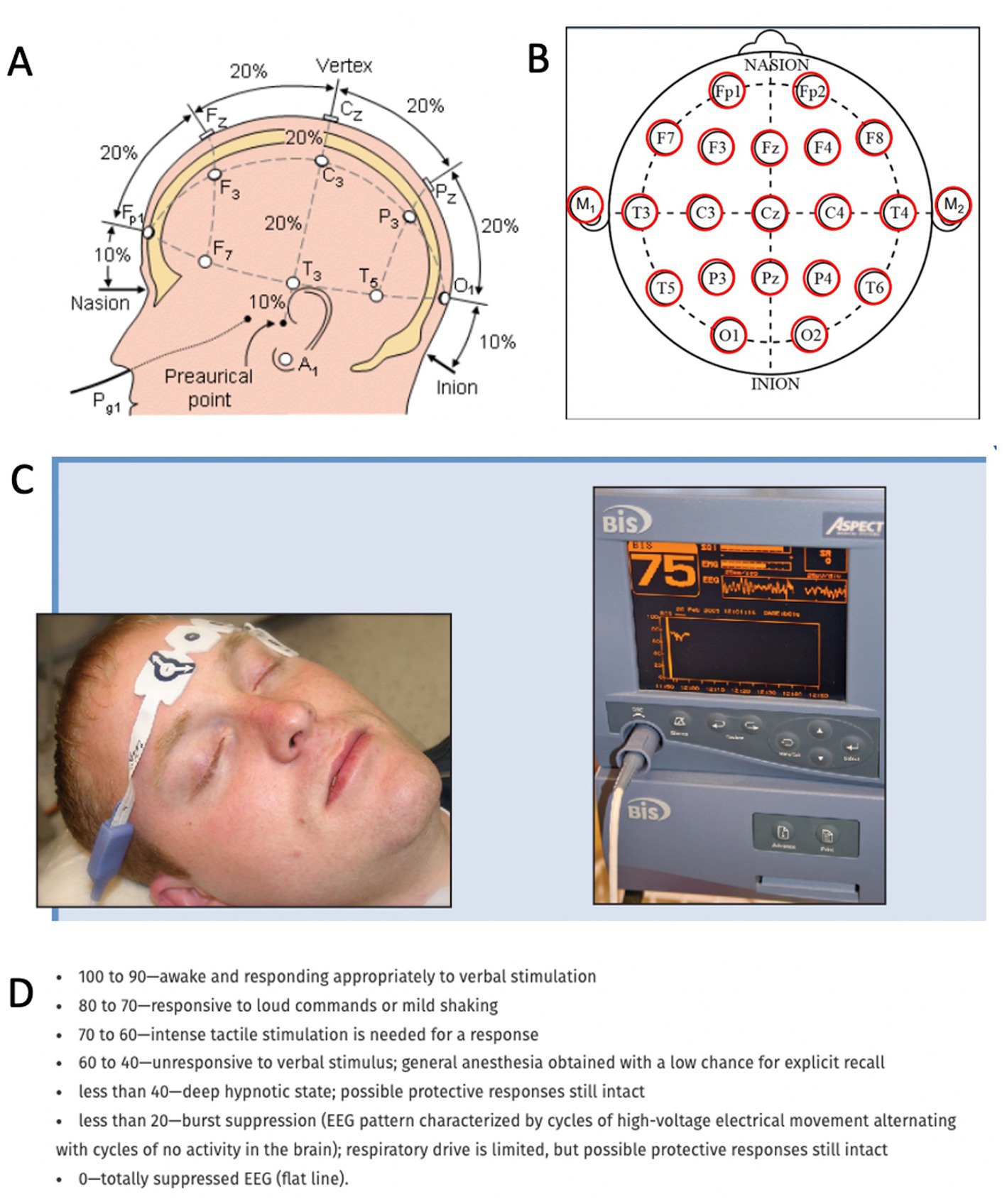The diagram features a comprehensive view of a medical procedure with four distinct sections, each with a scientific focus. In the upper left-hand corner (Image A), a side profile of a head illustrates anatomical landmarks and measurement percentages: the nasion at the front of the eyes, the inion at the back of the head, and the vertex at the top. Intervals of 10% and 20% are marked along the head's contour, including intra-cranial points like A1 near the ear, referred to as the pericardial (preauricular) point. 

Adjacent to it, in the upper right (Image B), is a concentric circle diagram representing the head from a top-down perspective. The diagram is anchored by the nasion at the top and the inion at the bottom, with M1 and M2 on the left and right sides, respectively. This grid, with labeled sections such as FP1, F7, F3, C3, P3, O1, PZ, and more, simulates the location of electrodes used in brain mapping.

The lower left quadrant features a photograph of a man with short blonde hair lying down with medical equipment attached to his head, seemingly undergoing a procedure. This equipment includes a head strap and electrodes positioned over his frontal lobe. 

In the lower right, there is an image of a computerized monitoring device displaying a reading of 75 in orange on a black screen within a gray unit labeled BIS and ASPECT. 

Finally, the text block in section D provides a detailed description of levels of consciousness and responses to stimulation, ranging from 100 to zero. It outlines different states from full awareness (100-90) to total EEG suppression (0), noting responses required at each level: from responding to verbal stimulus at higher levels to unresponsive states requiring intense tactile stimulation at lower levels, along with descriptions of general anesthesia and deep hypnotic states.